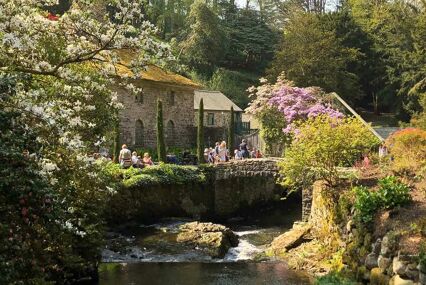The image appears to be a detailed painting of a serene landscape featuring a rustic setting with a house and a bridge. On the left side, a large tree adorned with numerous white flowers frames the scene. The focus shifts to a charming brown house with a mossy roof; it appears two to three stories high, with two upper windows and two arch-shaped entrances on the lower floor. In front of this house, people of all ages--men, women, and kids--gather, adding a lively human element. A stone bridge stretches in front of the house, with a river flowing beneath it, complete with a noticeable rock in its center. To the right, the landscape continues with vibrant pink and purple flowers, lush green leaves, and various trees, including mint and yellow ones. The background is filled with tall, imposing trees, enhancing the natural beauty of this picturesque setting.